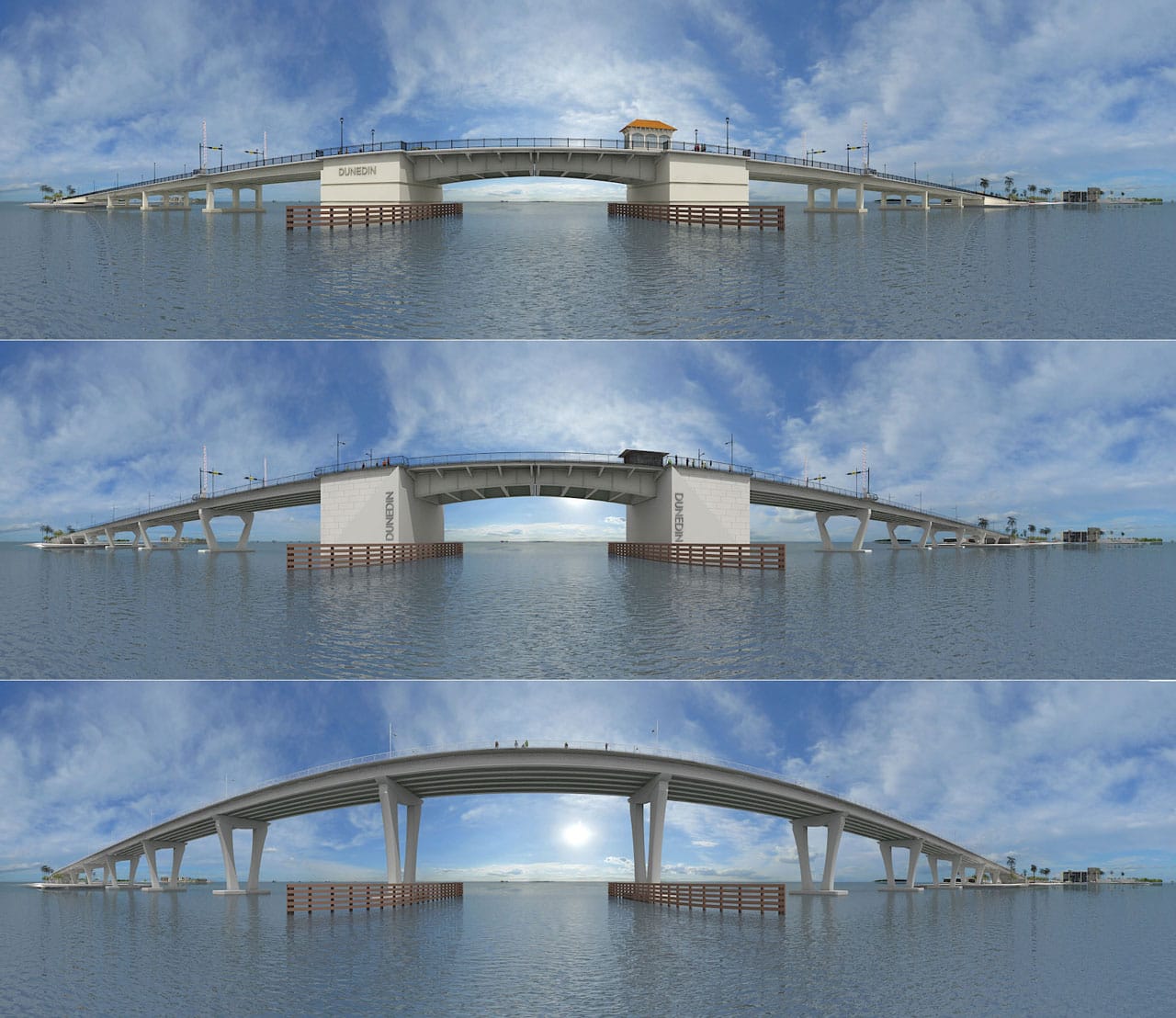The image is a panel featuring three distinct photographs of bridges, each showcasing a different bridge design and style over a body of water. The bridges are positioned vertically within the frame. The top photograph depicts a smaller bridge closer to the water with a low arc and a slight curve. The middle image shows a slightly taller bridge with a higher arc and taller pillars; it lacks a toll booth structure seen in other bridges. The bottom photograph highlights a very high, arched bridge with a prominent upward curve and thin, numerous supporting legs, offering a stunning overview of the water below. The color palette across the images includes shades of sky blue, white, grayish-white, brown, orange, and black, with a sky filled with blue and white clouds and blue water visible at the forefront.